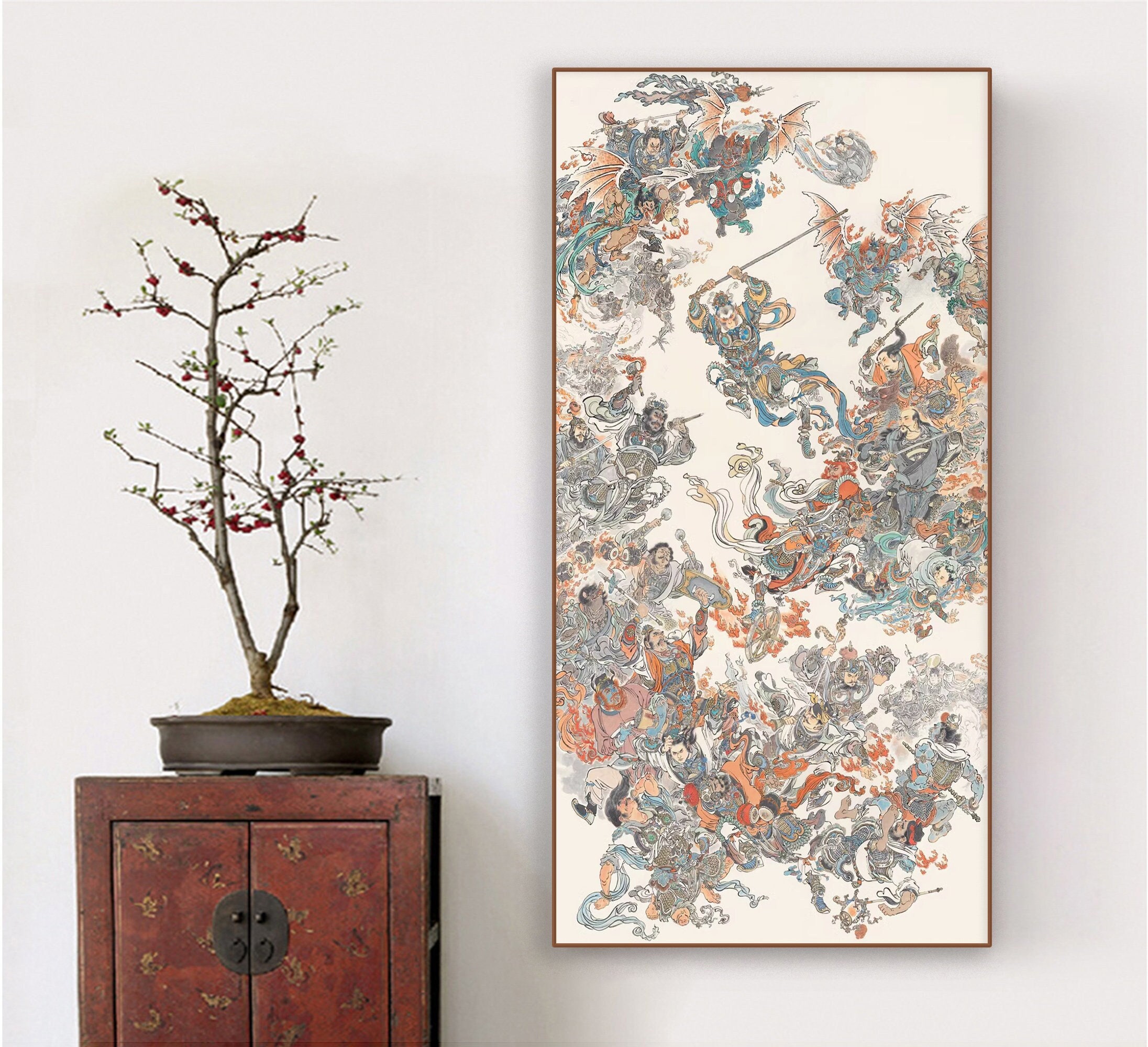This photograph, set against a stark white background, features two distinct objects. On the left side of the image stands a beautiful brown wooden chest with an ornate, possibly oriental design. This chest has two cabinet doors with a distinctive gray, oval-shaped plaque serving as the cabinet openers in its center. Atop the chest sits a dark brown round container holding an Asian plant that appears to be about two feet tall, with two branches adorned with berries on thinner branches. 

On the right side of the image, mounted against the white wall, is a rectangular painting that is taller than it is wide. The painting features a muted color palette of light aqua and rust, with some blues and reds. The abstract artwork depicts an array of Asian figures, including several samurai soldiers. In addition, there's a central figure holding a pole or a long sword, surrounded by various designs, including dragons and a flying creature with bat wings. This artful piece integrates a mix of scenes and features in a somewhat futuristic or abstract style.